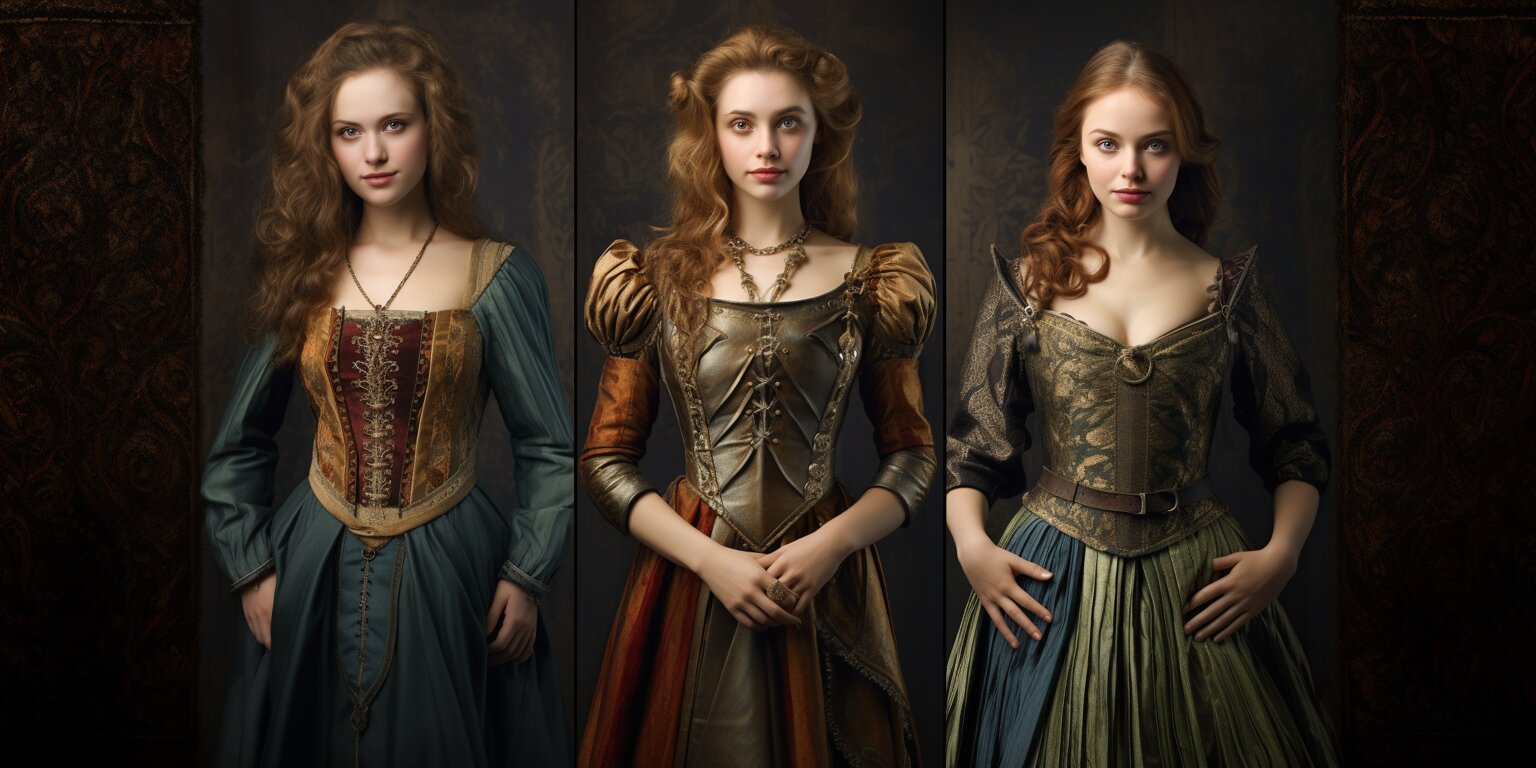This image is a triptych featuring the same woman in three different outfits, each reflecting a historical or fantasy aesthetic with a consistent dark wooden background. In all three images, the woman has long, wavy, reddish-brown hair styled slightly differently in each frame. 

In the first image on the left, she wears a dress with long green sleeves and a green skirt. The bodice features a pale yellowish print with a reddish center panel adorned with gold embroidery. She accessorizes with a brown necklace, and her hair falls forward on her right side. 

In the center image, her attire changes to a dress with puffy shoulder sleeves that transition to a tighter fit in shades of browns and rusts. The skirt is rust-colored with brown strips, and the bodice appears almost leather-like. She wears a choker necklace as well as a longer necklace extending into her dress, with her hands clasped together in front of her.

In the third image on the right, she wears a dress with three-quarter length bronze-colored sleeves and a green skirt embellished with blue on the right side. The bodice sharply tapers to a V-shape, revealing some cleavage and is cinched with a brown belt. Her hands are placed against her hips, revealing only three fingers and a thumb on her right hand.

This detailed portrayal emphasizes her historical costumes, distinctive hairstyles, and the subtle variations in her appearance across the three images.